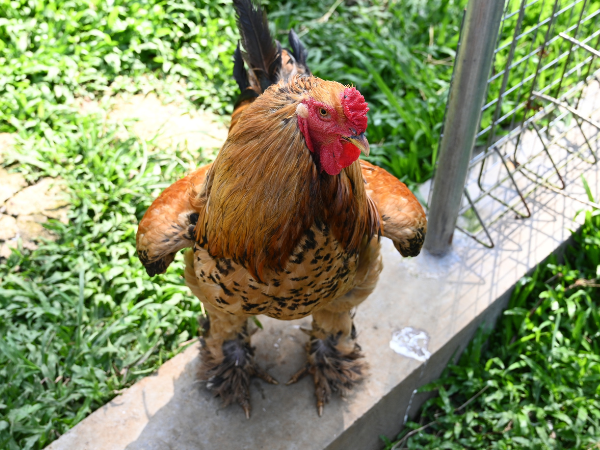This image captures a close-up, top-down view of a female chicken standing on a concrete slab surrounded by patches of green grass. The bird exhibits predominantly brown feathers, interspersed with black speckles, and darker brown and black-spotted plumage covering its feet. The chicken's wings are slightly spread, possibly to cool itself, revealing darker brown feathers with light brown centers and black tips. Around its neck, the feathers are darker brown and get progressively darker toward the body. The chicken, which also features a red skin flap on its chin and atop its head, is giving an intense, almost angry stare directly at the camera, adding to the image's unique character. Toward the back of the slab, there's some sort of wiring, potentially part of a fence or rack. Despite the bird's plump appearance and somewhat awkward stance, which might make one question the image's authenticity, the intricate details in the feathers and the setting contribute to a vivid and striking visual.